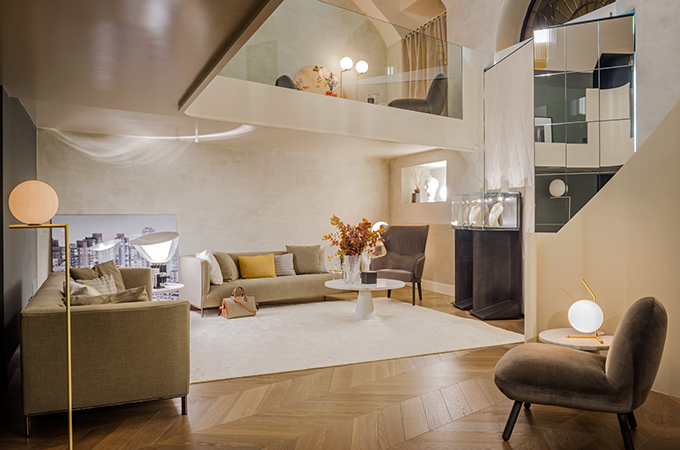This image showcases an elegant, high-class living room, likely in a house valued between $800,000 to $900,000. The room, adorned with beige walls, features two prominent beige sofas adorned with numerous throw pillows in shades of yellow, white, beige, and gray. At the bottom left corner, there is a solo armchair beside a green loveseat or ottoman. A luxurious Louis Vuitton handbag is casually placed on the pristine white carpet beside a white, round coffee table with a flower pot on it, slightly off-center in front of one of the sofas. The room is well-lit with various lamps, including a small globe-style lamp on a side table and a standing globe lamp adjacent to one of the sofas. There are two brown chairs angled at the sides of the room, a low-set velvet chair without arms, and a matching velvet wing chair with arms in the opposite corner. Display cases with internal lighting line the walls, accompanied by wall art depicting a cityscape. A balcony with clear glass railings overlooks the living room, adding an airy, open feel and flaunting more seating, curtains, and additional lighting above.